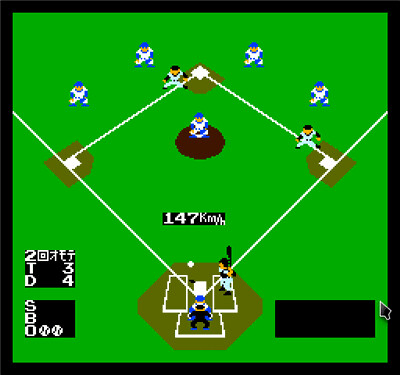This image is a screenshot from an old electronic baseball video game, reminiscent of an Atari game. The display is a square, mostly dominated by a bright green background representing the grass, but it's plain without any texture and bordered in black. The diamond layout is clearly depicted with white lines outlining the bases, home plate, and pitcher's mound. The bases and home plate are indicated by small brown diamonds, adding contrast to the green field.

Around the diamond are pixelated figures representing the players. The team in blue and white is in the field, and the team in black and white is at bat, with runners positioned on first and second base. Notably, there is a pitcher in white with blue details and a blue hat standing on the mound, and an umpire dressed in blue behind the batter, who is in a white uniform accented with a black belt.

The game's simplicity is evident in the visual details, such as the lack of grass texture and the rudimentary player animations. Additionally, a pitched ball is visible, traveling at a speed of 147 kilometers per hour. On the bottom of the screen, two black squares display game statistics and scores; one shows the scores for the 'T' team and 'D' team, which are 3 and 4 respectively, along with the count of 2 outs. The other black square lacks descriptive details but contributes to the nostalgic feel of this vintage baseball video game.